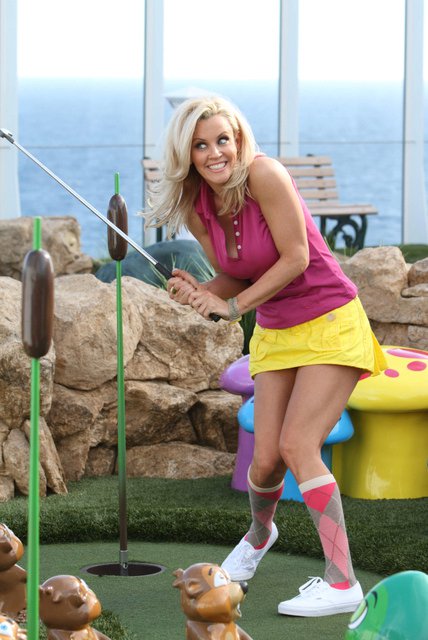Jenny McCarthy is captured mid-swing on a picturesque golf course, donned in a vibrant yellow skirt and a striking purple top. She completes her sporty look with knee-high golf socks and pristine white shoes. The putting green she's at seems to have the whimsical chaos reminiscent of "Caddyshack," with a multitude of gophers around the hole. The background reveals a serene ocean view under a white sky, and a bench placed thoughtfully to take in the scenery. Adding to the colorful landscape, golf sticks with what appear to be grapefruits are scattered around. The area is dotted with rocks, enhancing the rugged charm of the course. Jenny's knees are bent inward, showcasing her focused golfing stance.